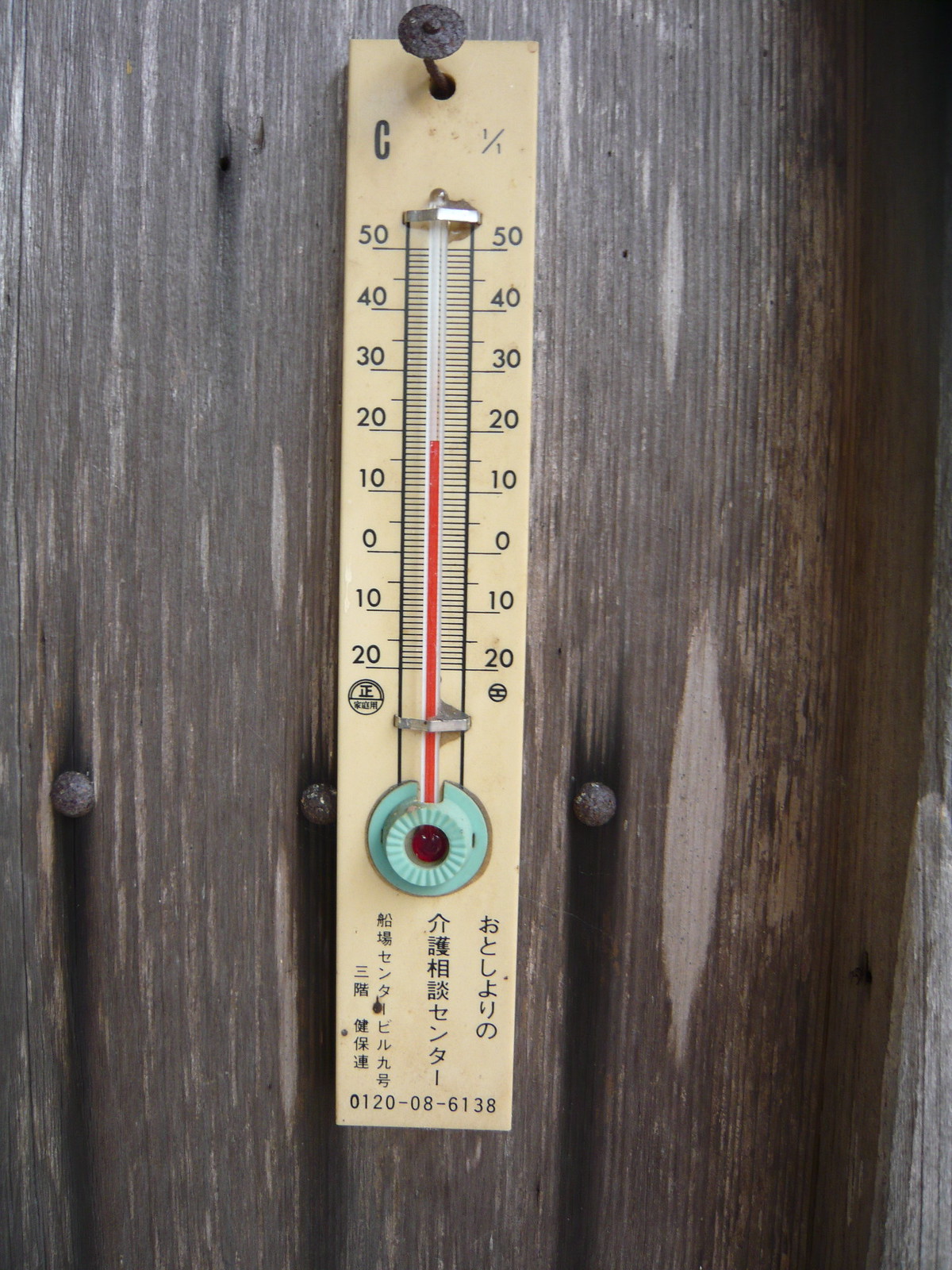A close-up photograph captures an outdoor thermometer mounted on a weathered wooden surface, likely a fence or wall. The wood, aged and darkened with time, is embedded with visible bolts on either side of the thermometer, enhancing the rustic aesthetic. The thermometer itself is cream-colored and features a turquoise plastic ring around its base, along with a turquoise circle encircling the adjustment knob. The mercury in the thermometer is rising, indicating a temperature of approximately 18 degrees Celsius. The temperature scale is clearly marked with black numbers on both sides of the thermometer. Below the turquoise knob, there is an inscription in Chinese, accompanied by a sequence of numbers along the bottom edge of the thermometer. The entire scene evokes a sense of nostalgia and resilience, highlighting the enduring functionality of simple, analog tools.